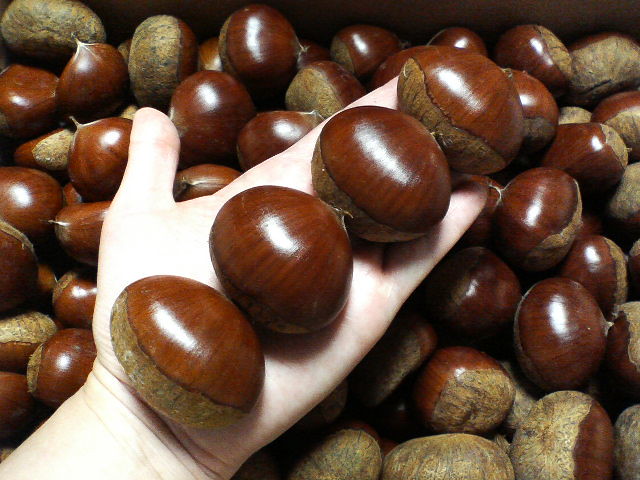The overhead photograph showcases a person's pale left hand, holding four abnormally large, shiny chestnuts, which fit snugly from their wrist to the tip of their fingers. These chestnuts display a rich, wood-brown color with clear stripes on their glossy tops and a light brown, dusty portion at the bottom, indicative of where they might have been attached to their shells. The background consists of a full box of similar chestnuts, adding a sense of abundance to the image. The well-lit, reflective shells contrast with the slightly obscured vertical dark surface at the top, suggesting the edge of the container they're in.